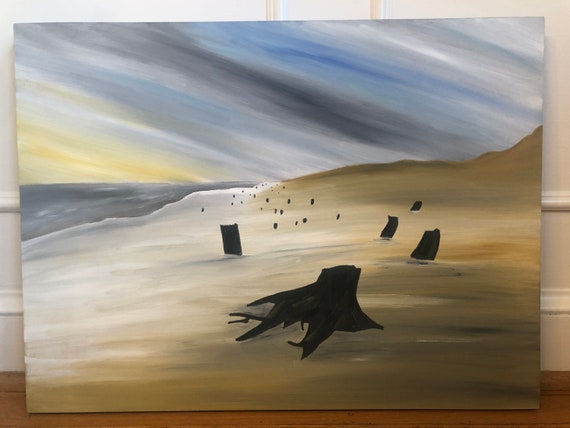The image appears to be a large photograph of an abstract painting that depicts a beach scene. The painting, unframed and on canvas, leans against a cream-colored wall with white molding and wooden wainscoting. The floor beneath it features wooden floorboards. Central to the image are tree stumps, some with visible roots, scattered along a beach comprised of murky yellow and green hues. The left side of the painting shows gray water transitioning to lighter, milky-colored sand near the shoreline. The sky above the beach is a tumultuous blend of stripes containing black, blue, white, and gray, with hints of yellow and orange, suggesting a stormy atmosphere or a time of transition like sunrise or sunset. The sky’s complex pattern and the scattered dark figures contribute to the painting’s abstract nature.